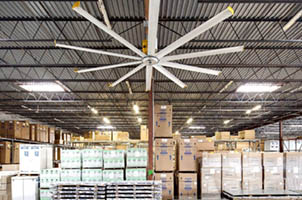Inside the expansive warehouse, numerous packages and boxes are meticulously stacked, reaching impressive heights. The boxes, predominantly brown and white, with some featuring light green accents, rest on both wooden pallets and metal shelving units. Overhead, the warehouse ceiling is composed of corrugated gray steel, supported by black metal beams running horizontally. Dominating the scene is a large industrial-sized ceiling fan with long, white blades extending from a central hub. Surrounding the fan are several bright, white square panel lights, illuminating the entire space. Additionally, a wooden post is visible amidst the storage. The intricate arrangement of packages, pallets, and the prominent ceiling features underscore the vastness of this organized warehouse interior.